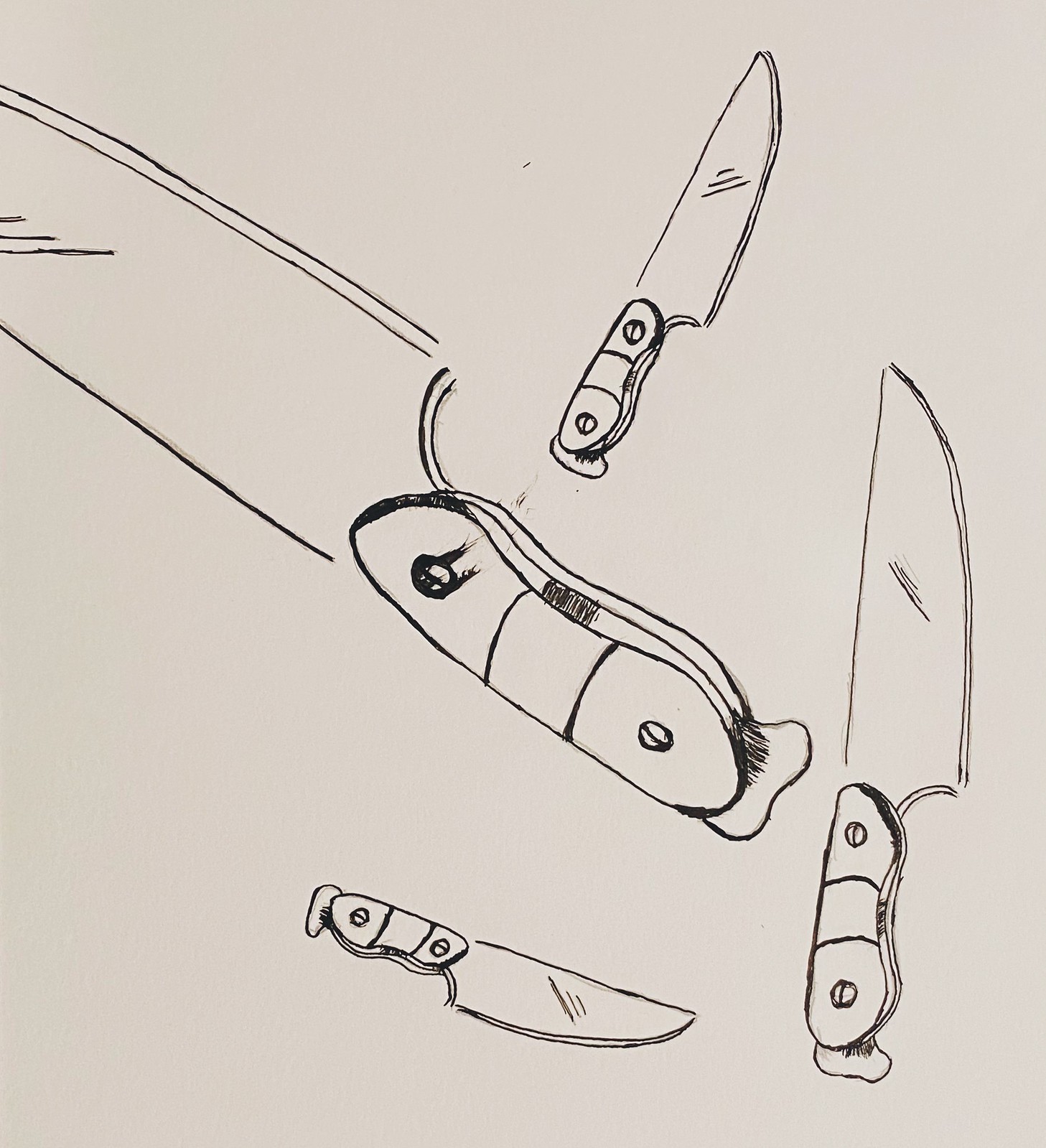This detailed black-and-white sketch showcases a collection of four knives, meticulously drawn and positioned at various angles. The centerpiece is a prominent, large butcher knife, diagonally oriented with its blade pointing upwards to the left. Its handle, secured with two screws and possibly fashioned from metal or acrylic, features a consistent curved wave design. Surrounding this central knife are three smaller knives, which share the same design — flat on one side with a pointed, curved blade. 

1. On the right side of the sketch, one knife stands vertically with its blade facing to the right.
2. Below the large butcher knife, another smaller knife lies mostly horizontal with the blade pointing right.
3. The final smaller knife lies diagonally, tip extending upwards to the top right, slightly above the large butcher knife. 

There are smudges throughout the page, suggesting this image was likely taken from an artist's practice sketchbook, capturing a detailed study of knife designs.